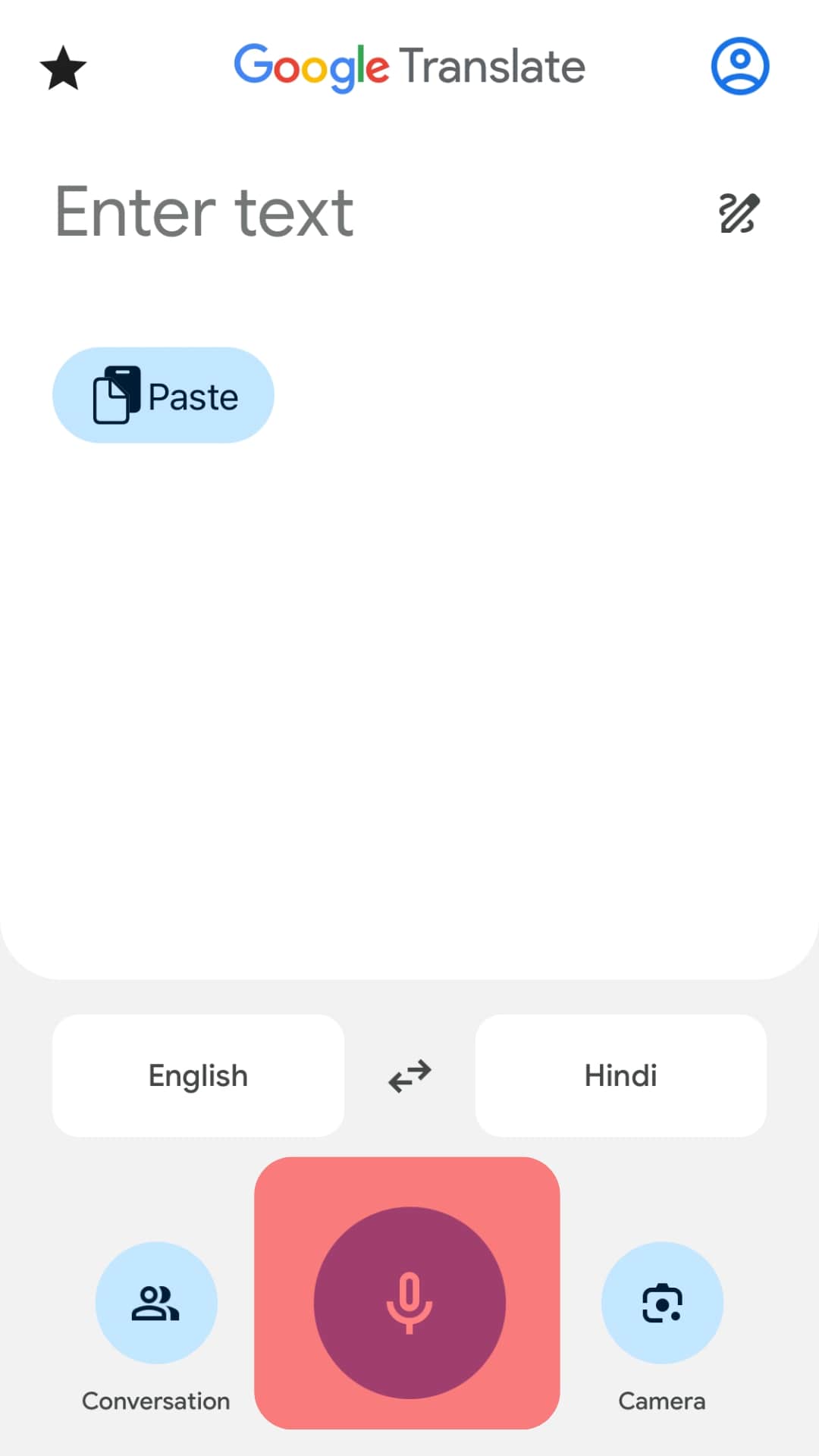This is a detailed screenshot of a Google Translate interface. At the very top, the screen prominently displays the heading "Google Translate." Below this title, there is a blank text box labeled "Enter text," inviting users to input text they wish to translate. Adjacent to this box is a blue icon labeled "Paste," allowing users to easily paste text.

Below this section lies a vast white space, presumably intended to display translation results once the input is processed. Further down, the active language translation pair is visible, which in this case is set to translate from English to Hindi. Users can select their desired source and target languages in this section.

At the very bottom of the interface, there is a large red microphone button, designed for voice input. This button enables users to speak the text they want to be translated, which will then be converted into the chosen language. To the right of the microphone button, there is a camera icon, likely intended for translating text captured through the device's camera.

To the left of the voice input button is a conversation icon. This feature presumably allows multiple users to join a conversation, facilitating real-time multilingual communication.